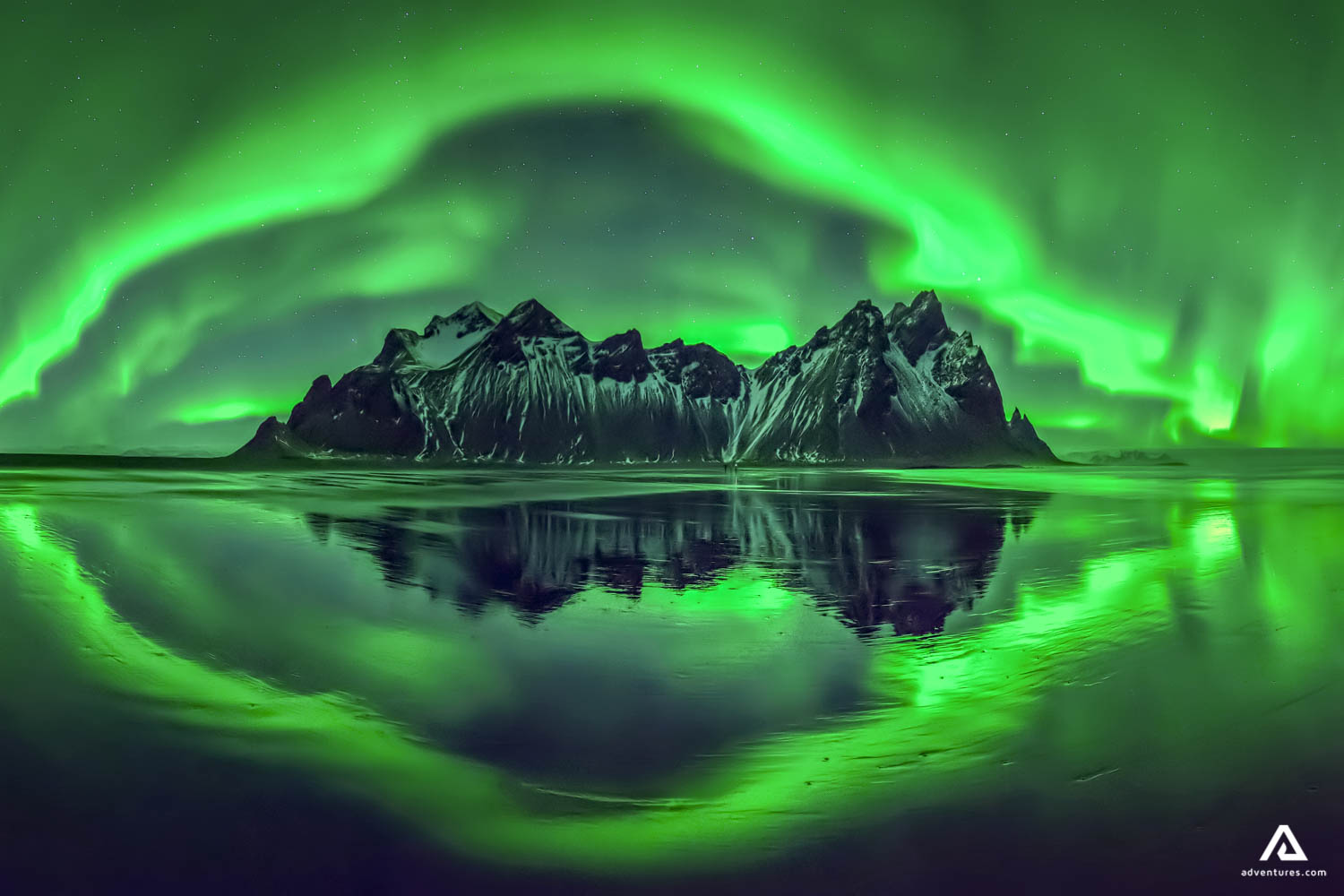In this highly detailed and surreal illustration, a black, rocky mountain formation stands majestically at the center, surrounded by a frozen lake. The scene, illuminated by a dramatic display of the Aurora Borealis, features vivid green ripples and waves that dominate the sky, casting a luminous glow upon the landscape. The green hues are reflected in the smooth, mirror-like surface of the lake, creating a symmetrical double image that enhances the surreal atmosphere. The sky exhibits a variety of green shades, forming a large, captivating oval. Below this entrancing natural phenomenon, the image has a logo in the bottom right corner showcasing a stylized "A" with the text "ADVENTURES.COM" beneath it. Although the environment appears otherworldly, possibly resembling a scene from a video game or artwork, the meticulous details and symmetrical reflections add a layer of realism that bridges the gap between imagination and reality. No people, animals, or buildings are visible, emphasizing the pristine and undisturbed nature of this fantastical landscape.